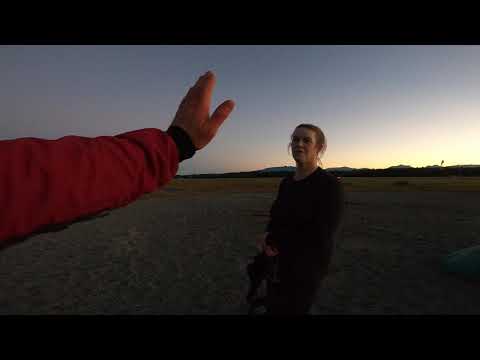This horizontally aligned rectangular photograph, bordered with thick black bands at the top and bottom, captures what appears to be a moment of tension or significant interaction as evening approaches. The sky overhead is a darkening blue transitioning to bright white near the horizon. Central to the image is a woman with brown hair tied back in a ponytail, dressed entirely in black attire. Her expression suggests a mix of contemplation and hesitation as she faces a man whose extended left arm is visible on the left side of the frame. His hand, palm up, appears to signal her to stop. He wears a red long-sleeve jacket or sweatshirt with a black cuff. The ground they stand on seems to be a drab, brownish-gray mix of dirt or sand. Sparse, green grass is visible in the background, along with slight hills and a strip of trees lining the horizon, all under the dimming twilight sky.